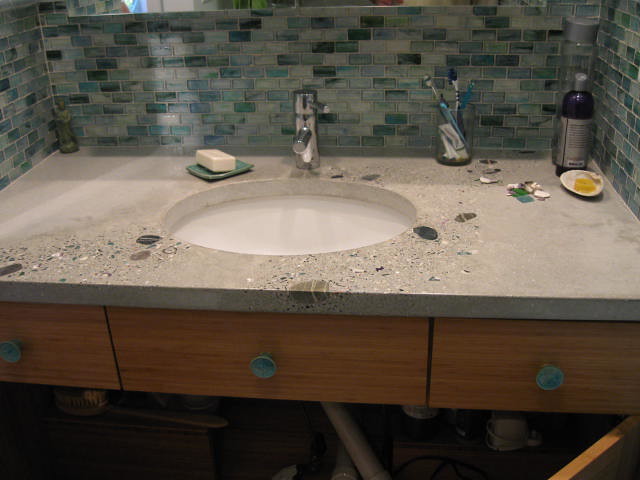Indoor close-up photograph of a bathroom sink featuring a natural stone or concrete countertop with an under-mount white porcelain basin. Below the countertop are three wooden drawers, each adorned with a simple circular pull in the center. Positioned on the countertop behind the sink is a sleek, chrome single-handled faucet with a cylindrical, perpendicular nozzle. 

To the left of the faucet lies a flat green soap dish holding a pristine bar of white soap. On the right side, against the backsplash, there's a clear cup containing two toothbrushes, possibly accompanied by some toothpaste. In the far right corner, a clear container is visible with a shampoo bottle in front of it, its cap securely closed. An upside-down seashell with a yellow object inside adds a touch of the seaside to the scene.

The backsplash itself comprises a mosaic of small, rectangular tiles in various shades of dark blue, light blue, and teal. A hint of a mirror is seen in the upper left, bordered by what appears to be stainless steel, although the details are not very clear. The image suffers from poor lighting and is slightly out of focus, giving it a somewhat hazy appearance. No text or print is visible in the photo, maintaining the focus on the bathroom sink setting.